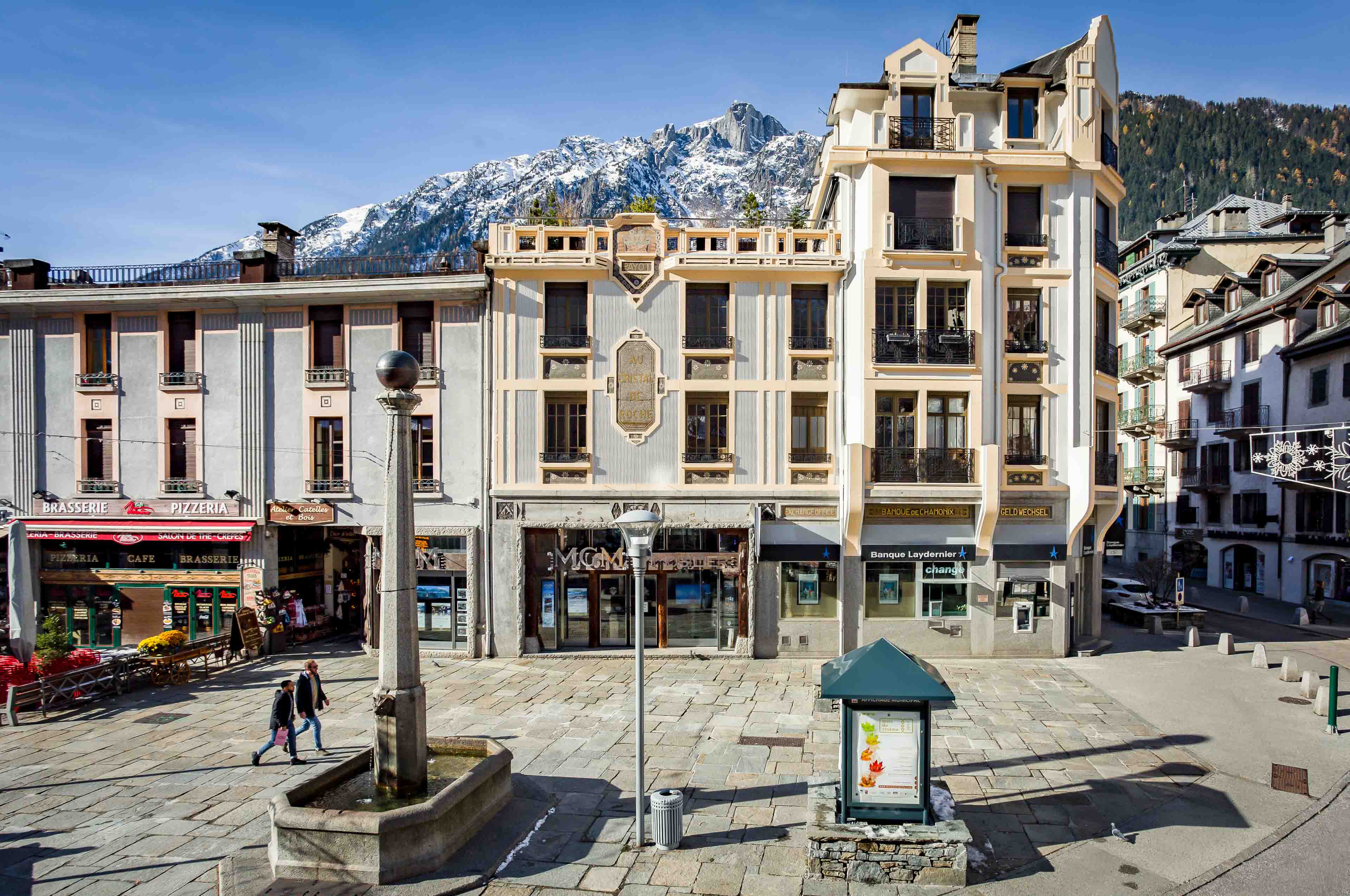This daytime photo portrays a bustling courtyard in an alpine village, framed by a stunning backdrop of clear blue skies and snow-capped mountains. The courtyard itself is paved with old tan stones, leading to a charming fountain with a pole crowned by a round metal ball, from which water flows into a small pool. Green benches adorned with yellow and pink flowers line the area, inviting passersby to sit and enjoy the picturesque surroundings.

Dominating the scene are several buildings with vintage architecture, featuring large vertical windows, balconies, and multiple floors. The ground level is lined with various shops, including a pizzeria with a small red overhang, and businesses with signboards displaying names like "Brazieri," "Crepes," "Saloon," "Dairy," "Atelier," and "MGM." The vibrant commercial zone also includes a movie theater labeled "MGM," contributing to the lively atmosphere.

In the foreground, benches, small plants, and flowers add to the courtyard’s charm, complemented by lampposts, dustbins, and hoardings. People walk along the pavements and cars are visible in the background, highlighting the area's dynamic energy as a hub of activity.